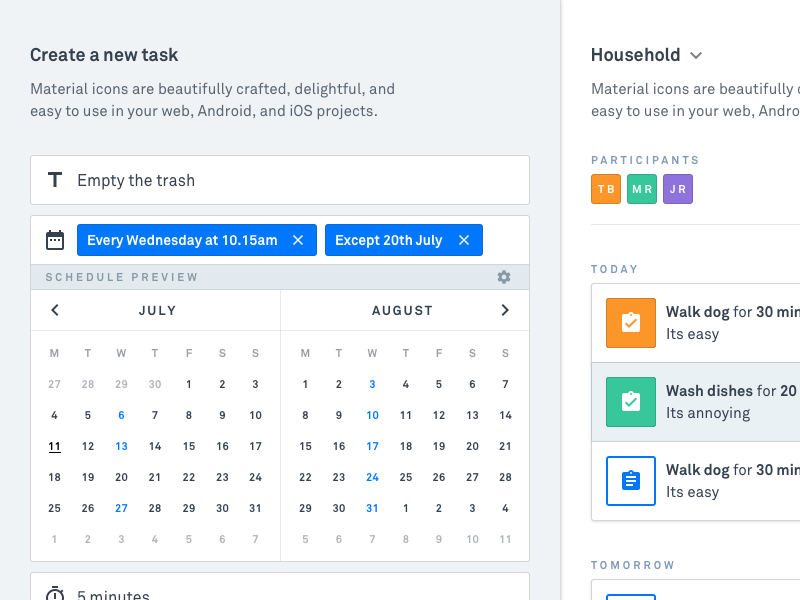This image is a detailed screenshot of a task management interface set against a primarily light gray background. At the top left of the screen, bold black text reads, "Create a new task." Directly beneath this, another line of black text, also in bold, states, "Material icons are beautifully crafted, delightful, and easy to use in your web, Android, and iOS projects."

Below this description, there is a white box containing the text "Empty the trash," followed by an icon for the calendar. Next to this icon, within a blue box, the text reads, "Every Wednesday at 10:15 a.m." Another blue box beside it adds, "Except 20th of July."

Further down, a gray banner spans the width of the screenshot, displaying the text "Schedule Preview" with a settings icon situated to the right of the text. To the left of the banner, there's a monthly calendar view for July and August. Dates are highlighted in blue, specifically the 6th, 13th, and 27th of July, as well as the 3rd, 10th, 17th, 24th, and 31st of August.